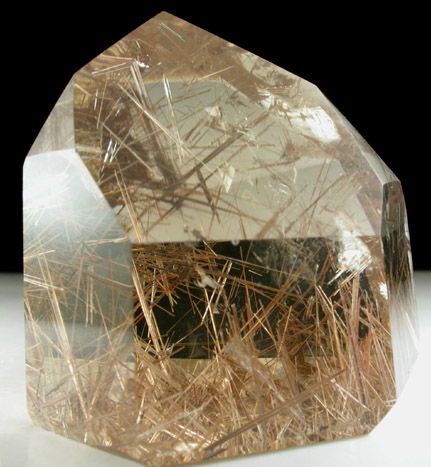The image shows a striking decorative crystal, possibly quartz, resting on a white platform against a completely black background. The crystal, resembling a jagged diamond shape, contains an intricate and busy pattern of hay-colored twigs or wood pulp embedded within its see-through, glass-like structure. The crystal's surface is marked by cuts and possibly reflections, which create an impression of additional twigs or hay surrounding it. The entire crystal segment, with its intricate details and distinctive coloration, appears to be carefully curated as a piece of art, potentially displayed in a museum setting.